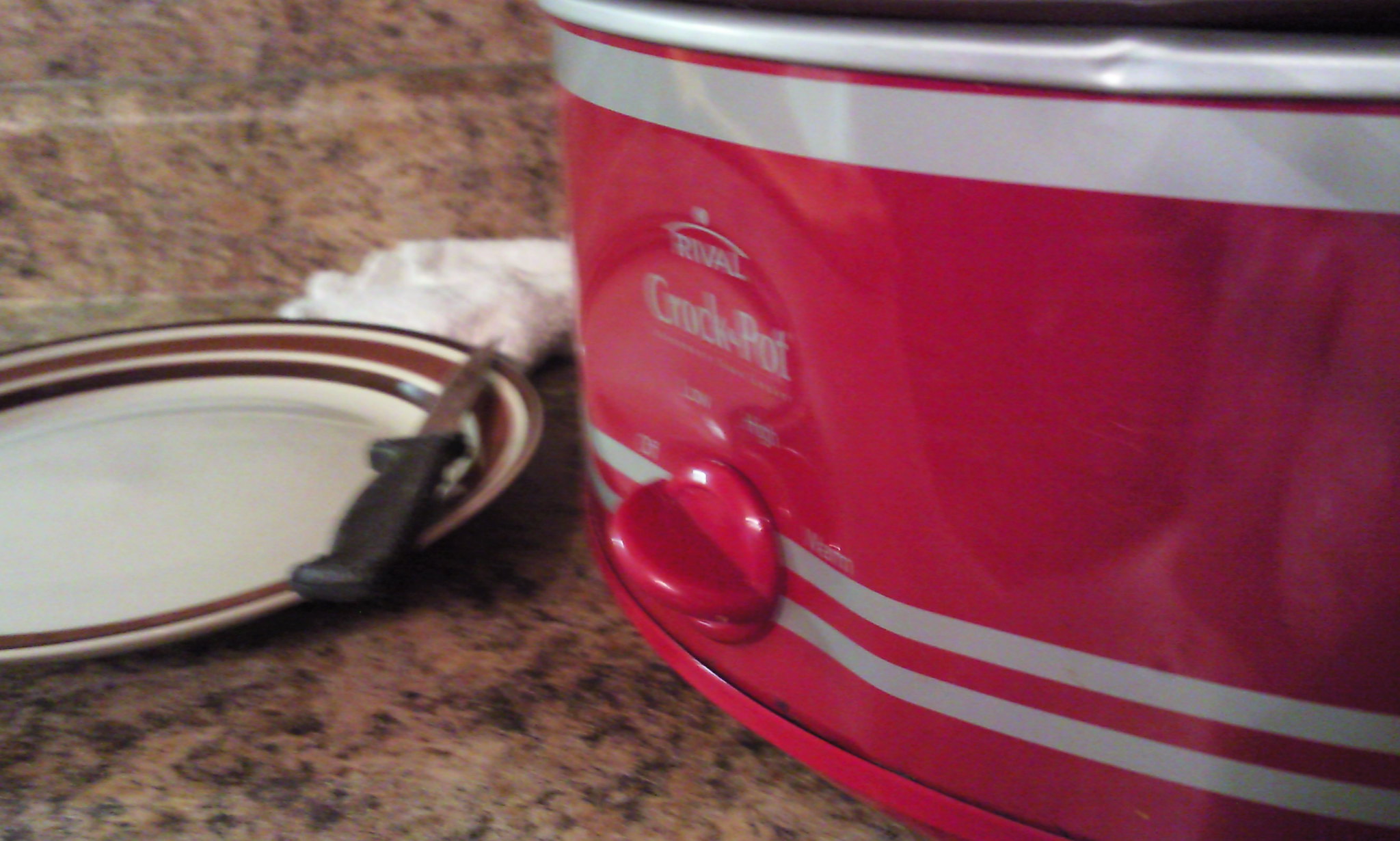This detailed color photograph features a cluttered kitchen countertop made of brown and black marble or granite. On the left, there is a ceramic plate with two or three brown stripes around the edge, and it is predominantly white in the center. Resting on the right edge of the plate is a black-handled, silver-bladed knife, possibly a paring knife. Behind the plate, a white napkin or towel is either crumpled or folded. Dominating the right side of the image is a red Rival Crock-Pot with two silver stripes at the bottom and one at the top, as well as a silver rim around the upper edge. The Crock-Pot's front is labeled with "Rival" and "Crock-Pot" in gray text. It features a large red knob with a gray stripe at the top, which allows the user to set it to one of four positions: Off, Low, High, and Warm. The photo is somewhat blurry, particularly around the text on the Crock-Pot, but these details stand out prominently.